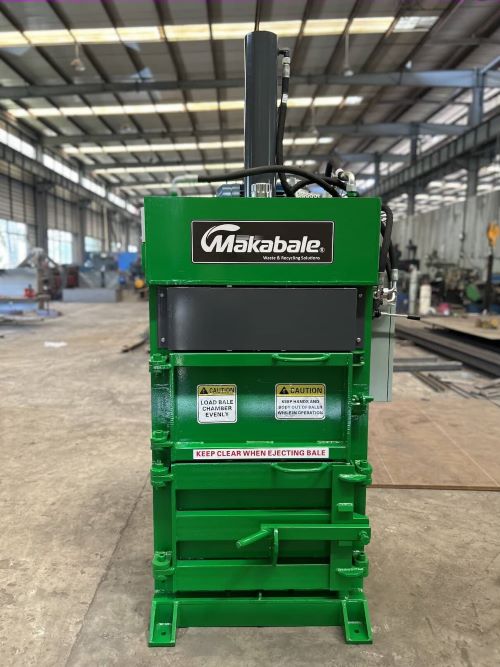The image depicts a green baler machine positioned centrally on a warehouse floor with a blend of wood and concrete, under a grey metal roof with extensive lighting. This machine, standing approximately four to five feet tall and reminiscent of the size of a vending machine, is prominently green with a black-bordered panel at the top displaying the brand name "MAKABALE" in white letters. Directly below, there's a solid black rectangle followed by two caution stickers. The left sticker reads "Load Bale Chamber Evenly" and the right sticker is partially legible with "Keep Clear When Ejecting Bale" in red on a white strip below it. The baler includes handles on each level and is positioned on green feet. The surrounding area features metal walls and various other devices, with a large piece of wood lying on the ground to the right and expansive garage doors allowing light to spill into the cement floor, which shows yellowish-brown spots.